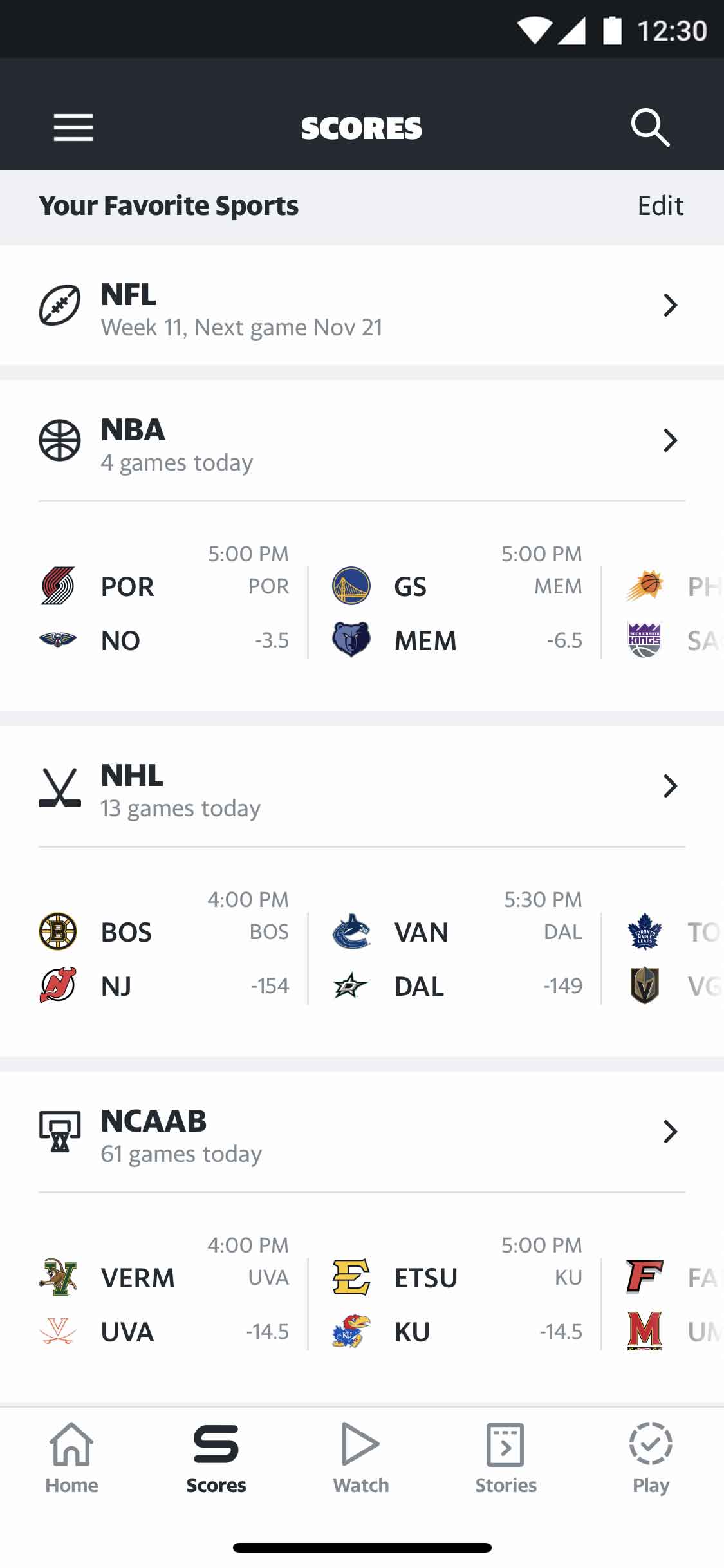The image is a screenshot taken from a smartphone. At the top of the screen, the phone displays a full Wi-Fi signal, full cellular bars, and a full battery, with the time of 12:30 shown against a black background. Beneath this, there is a section with a dark gray background featuring three horizontal white bars stacked on top of each other. The word "SCORES" is prominently displayed in white capital letters at the center, with a magnifying glass icon on the right side, suggesting a search function.

Below this, another dark gray box appears, labeled "Your Favorite Sports" in white text on a black background, with the word "EDIT" aligned to the right. The subsequent section has a light gray background listing various sports:

1. NFL - indicated by a football icon, it mentions "Week 11" and "Next game November 21st," with an arrow pointing to the right on the right side.
2. NBA - represented by a basketball icon, it displays "4 games today," accompanied by another arrow on the right side. Specific game details follow:
   - POR vs. NO at 5 PM, with NO favored by -3.5.
   - GS vs. MEM at 5 PM, with MEM favored by -6.5.
   
At the bottom of the screen, there is a box labeled "NHL."